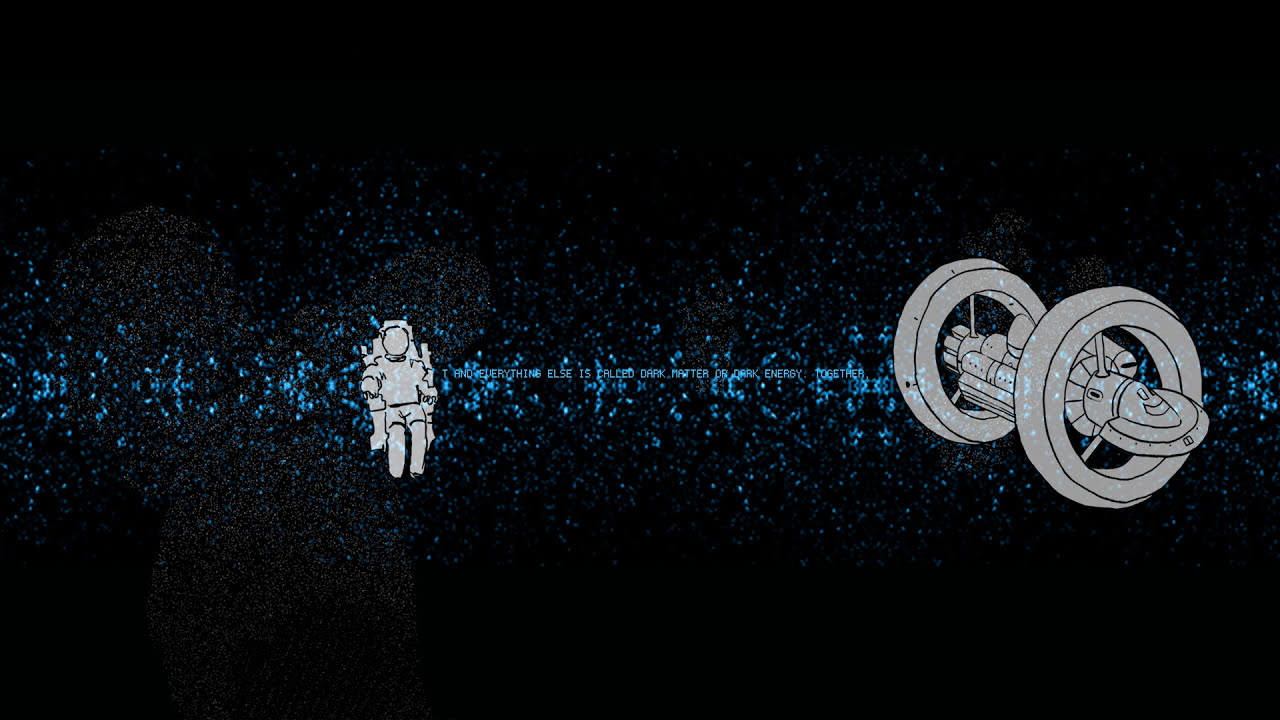The image is a cartoon-like digital artwork set in space, dominated by a primarily black background accented with bright blue sparkles resembling star dust. On the right side of the image floats a distinct, white or grey spaceship with a design featuring two attached circular structures, reminiscent of wheels, encasing what appears to be the shuttle or spacecraft's core. To the left of the spaceship, an astronaut, similarly colored in white or grey, drifts in the vastness of space, wearing a spacesuit and helmet. Between the astronaut and the spaceship, there's small, hard-to-read text in the same bright blue color as the star dust. The overall effect is a pixelated or digitalized aesthetic, capturing a scene teeming with a sense of cosmic wonder and the mysterious vastness of the universe.